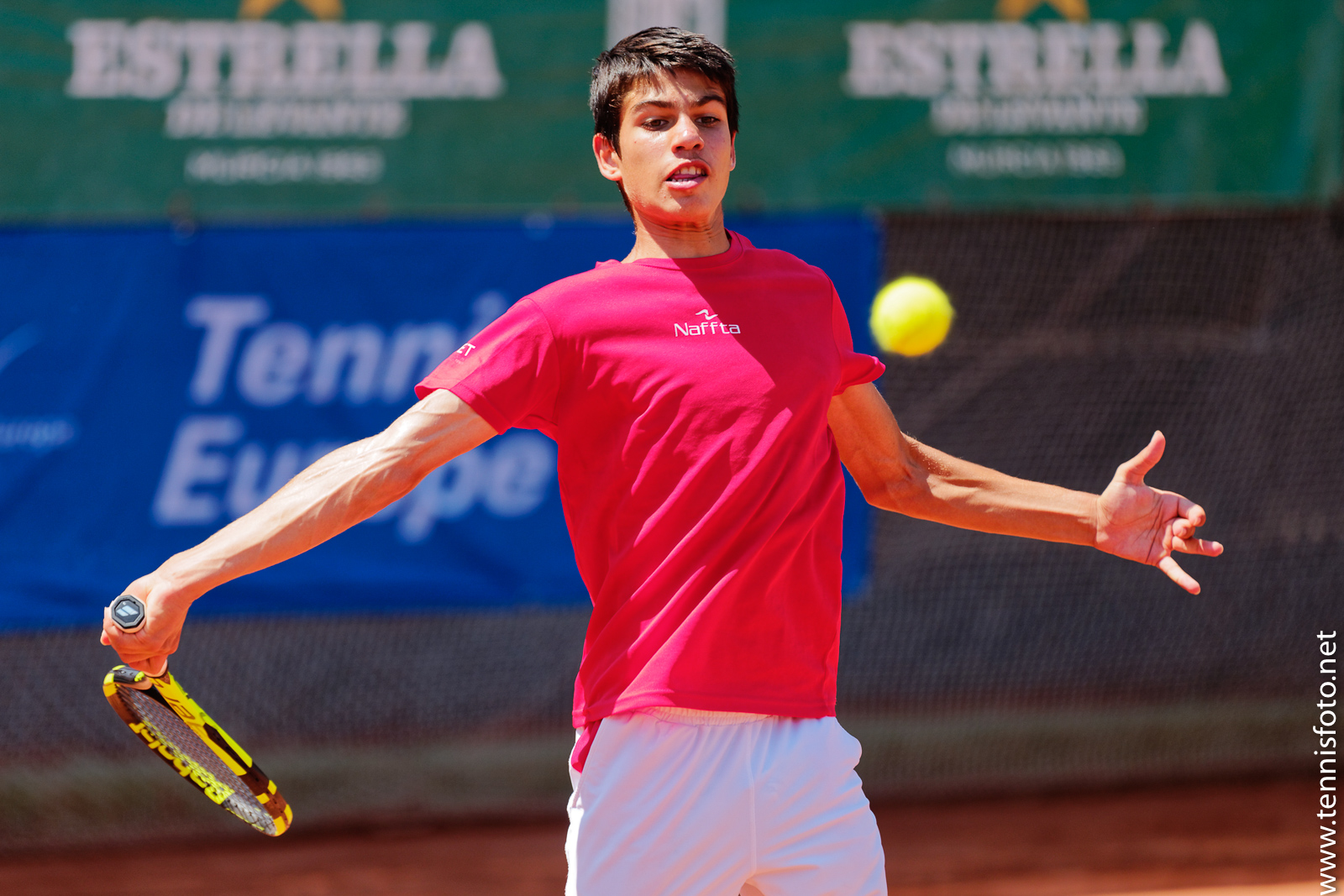The image showcases a young Caucasian male, possibly of Arabic descent, actively playing tennis on a court. He is focused intently on an incoming yellow tennis ball, preparing to hit it with a bright yellow and black Babolat racket held in his right hand. Dressed in a red t-shirt with white lettering and white shorts, the athlete is captured in a dynamic pose with his arm stretched back, ready to swing. The background features a fence adorned with banners: two green ones with the word "Estrella" in white, and a blue banner partially obscured by the tennis player, displaying "Tennis Europe" in white lettering.